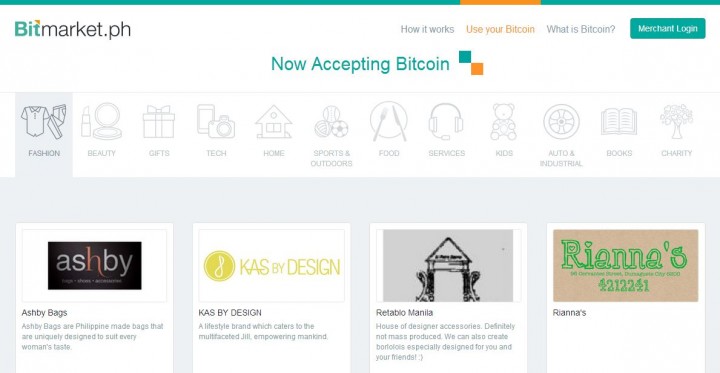This image is a cropped screenshot from the webpage Bitmarket.ph, with the browser details removed. The website's logo, located in the top left corner, reads "bitmarket.ph." In the top right corner, navigation menu options are visible, with "Use Your Bitcoin" highlighted in orange, indicating it as the selected option. A blue rectangle button for logging in is also present.

The webpage appears to be structured as a shopping platform. Various categories are displayed via icon-based line drawings representing different shopping sections such as fashion, beauty, gifts, food, kids, and books. The "Fashion" category is currently selected. 

Below the category icons, the "Fashion" section displays four rectangular white boxes. Each box includes a shop logo and a brief text description of the corresponding shop.